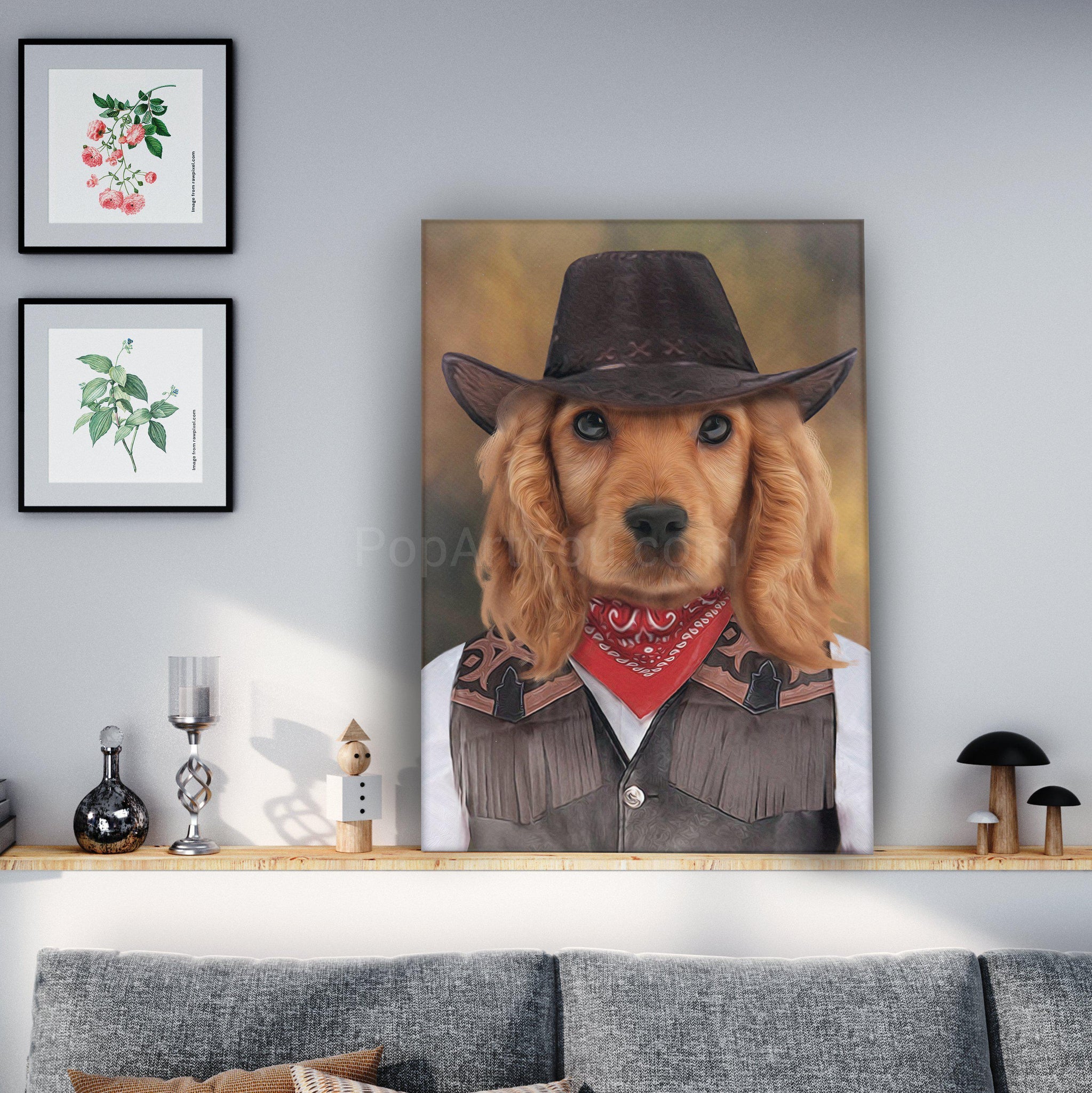In this image of a cozy living room, a prominently placed picture of a golden retriever or cocker spaniel dressed as a cowboy captures immediate attention. The dog, with its fluffy, drooping gold ears, big brown eyes, and black nose, sports a black cowboy hat adorned with brown X's on the headband, a red bandana around its neck, and a black leather vest over a white long-sleeved shirt. This charming picture is centrally located, directly above a gray couch that features two brown pillows on the right side. To the top left of the dog picture, two smaller, framed portraits hang, one depicting green leaves and the other showing pink flowers with green leaves, both in black frames. Below the portraits is a light brown wooden counter or baseboard, decorated with various objects including a silver candle, a silver vase, a wooden doll, and a mushroom carving. The light gray wall serves as a backdrop, contributing to the room's overall warm and inviting atmosphere.